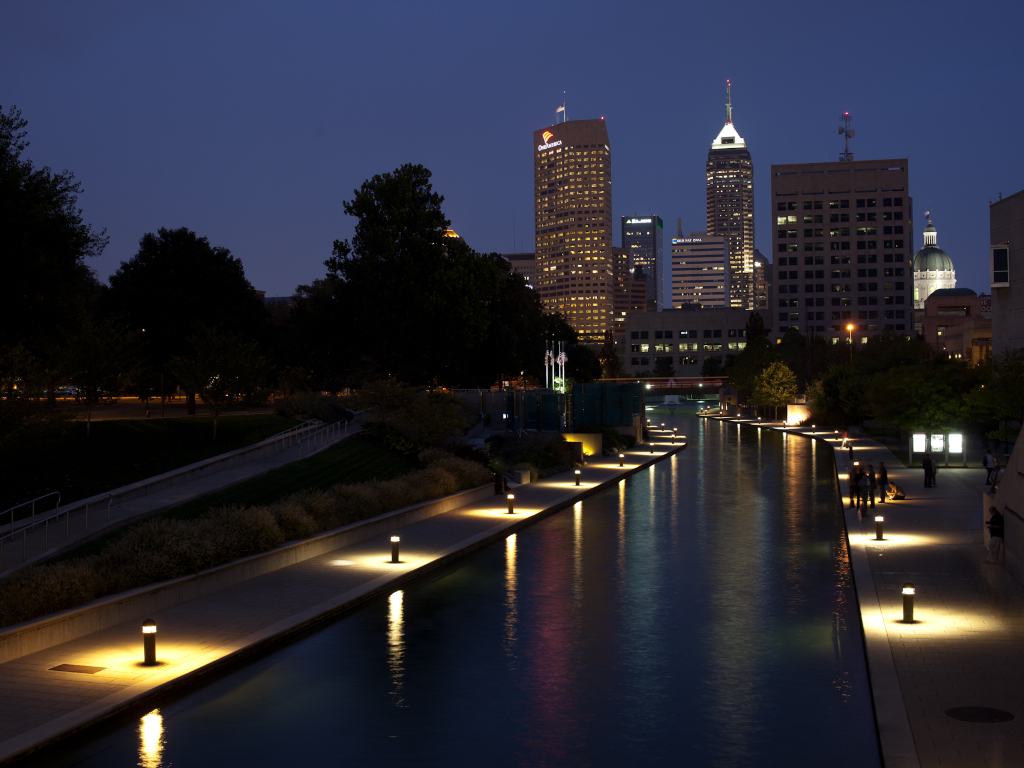This nighttime photograph captures a serene urban riverwalk scene. The image vividly portrays a narrow river running vertically through the center, flanked by concrete sidewalks on both sides that feature evenly spaced light sconces emitting a soft, round glow. Amidst the tranquility, a few silhouettes of people are visible, adding life to the scene. On the left side, a small park area can be discerned, characterized by the presence of large trees, their outlines stark against the clear, starless sky.

Above, the cityscape is dominated by tall, illuminated buildings, including a high-rise in the upper right corner and another on the left possibly bearing a slightly blurred "Bank of America" sign with an orange flag above it. Further along the river, it flows under a bridge that connects two buildings, suggesting a potential walkway or work area. The absence of clouds enhances the reflection of city lights on the river's surface, presenting a clear and calm atmosphere. The lampposts, lit-up signs, and the glowing skyline collectively paint a vibrant yet peaceful nocturnal portrait of the city's riverwalk.